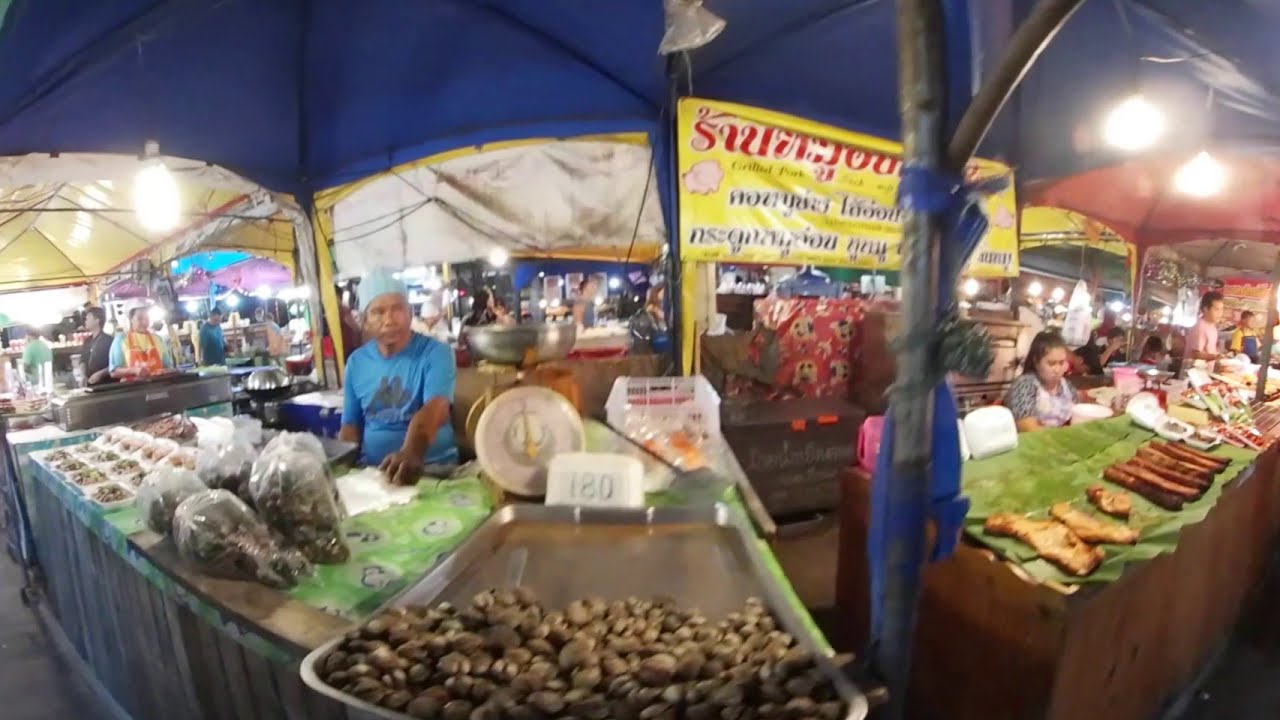The photograph captures a bustling, open-air market in a foreign country, taken with a fisheye lens, giving it a warped appearance. At the center of the image, a man in a blue shirt and a beanie stands under a blue canopy. In front of him is a green table covering adorned with images, laden with loose and bagged food items, possibly nuts or fish, and a set of scales. To his right, a woman wearing a black and white shirt with an apron offers what seems to be bread. On the left, other vendors are present with various food products displayed on bare plywood tables, also covered with green blankets. The market has a blue tarping roof with lights hanging from it. In the background, there is prominent yellow and red signage featuring text in a different language, with mentions of grilled pork, adding to the authenticity of this foreign marketplace. This scene is vividly alive with vendors and customers surrounded by an array of foods, indicating the cultural richness of this locale.